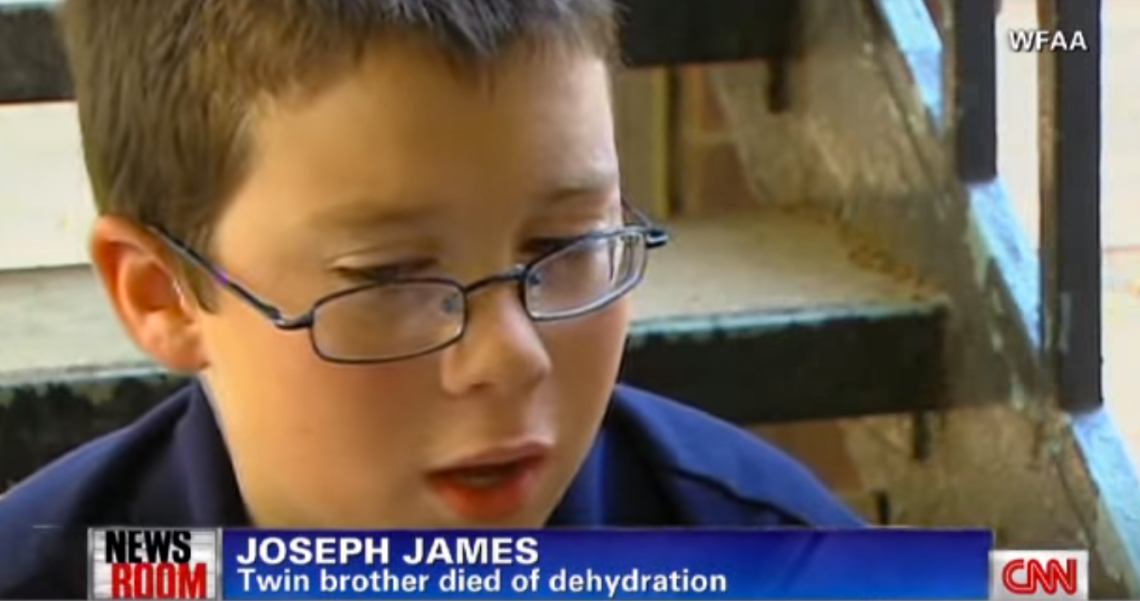The image depicts a still from a CNN news broadcast, as indicated by the red CNN label on a white background in the bottom right corner. The top right corner bears the white text "WFAA." Central to the image is a small boy, identified by the news caption as Joseph James. The boy, approximately 8 or 9 years old, has dark, brown hair and wears black-rimmed square glasses along with a blue shirt. He is seated at the bottom of an old staircase with black metal railings, looking downward and speaking, his mouth slightly open, giving off a somber demeanor. The news caption below his face reads: "Newsroom, Joseph James, twin brother died of dehydration," indicating the tragic loss of his twin brother.